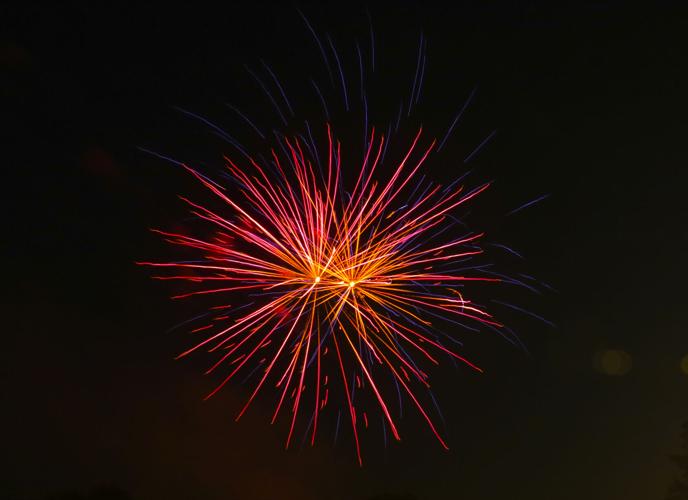The image captures a vibrant fireworks display against a pitch-black sky, showcasing a mesmerizing explosion of colors. At the forefront, two primary bursts dominate the scene. Each explosion radiates from a bright center—the first featuring a core of brilliant white that transitions to yellow, then to pink, and eventually deepening into hues of dark orange, yellow, and red. The second burst mirrors this pattern but integrates darker shades more pronouncedly, with outer streaks manifesting in deeper reds and oranges. There are notable blue streaks at the top, extending down and under the explosions, adding a cool contrast to the predominantly warm color palette. 

Interspersed among the main streaks are small red droplets, most of which descend towards the ground, highlighting the dynamic movement of the fireworks. Additionally, the background features subtle purple sparks that add depth to the display, and a distinct yellow lens flare appears at the bottom right, enhancing the image's overall radiance and complexity.